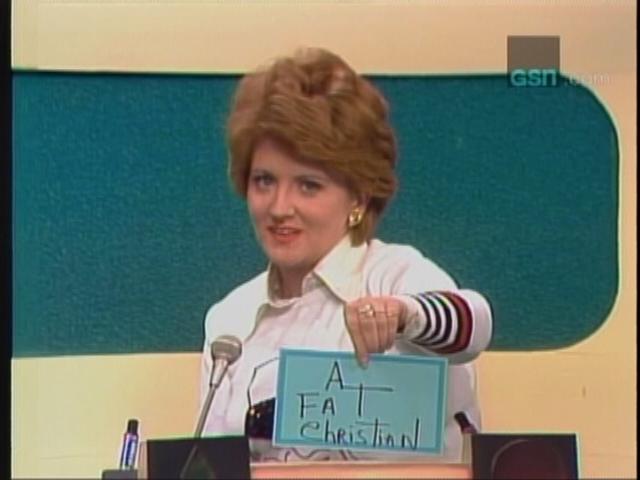The image portrays a vintage game show scene, evident from the GSN.com logo in the top right corner, indicating it is likely from the Game Show Network. The setting evokes a nostalgic vibe, possibly from the 70s or 80s. The background features a cream-colored wall with a distinct teal rectangle. The focal point is a woman in her 40s with medium-length, poofy dark brown hair and striking red lipstick. Her attire comprises a white sweater layered over a white collared shirt with striped sleeves. She accessorizes with gold earrings and a ring. Positioned at a podium or desk equipped with a silver microphone and a marker, she holds up a blue piece of paper with handwritten text that reads "a fat Christian," directly engaging with the camera.